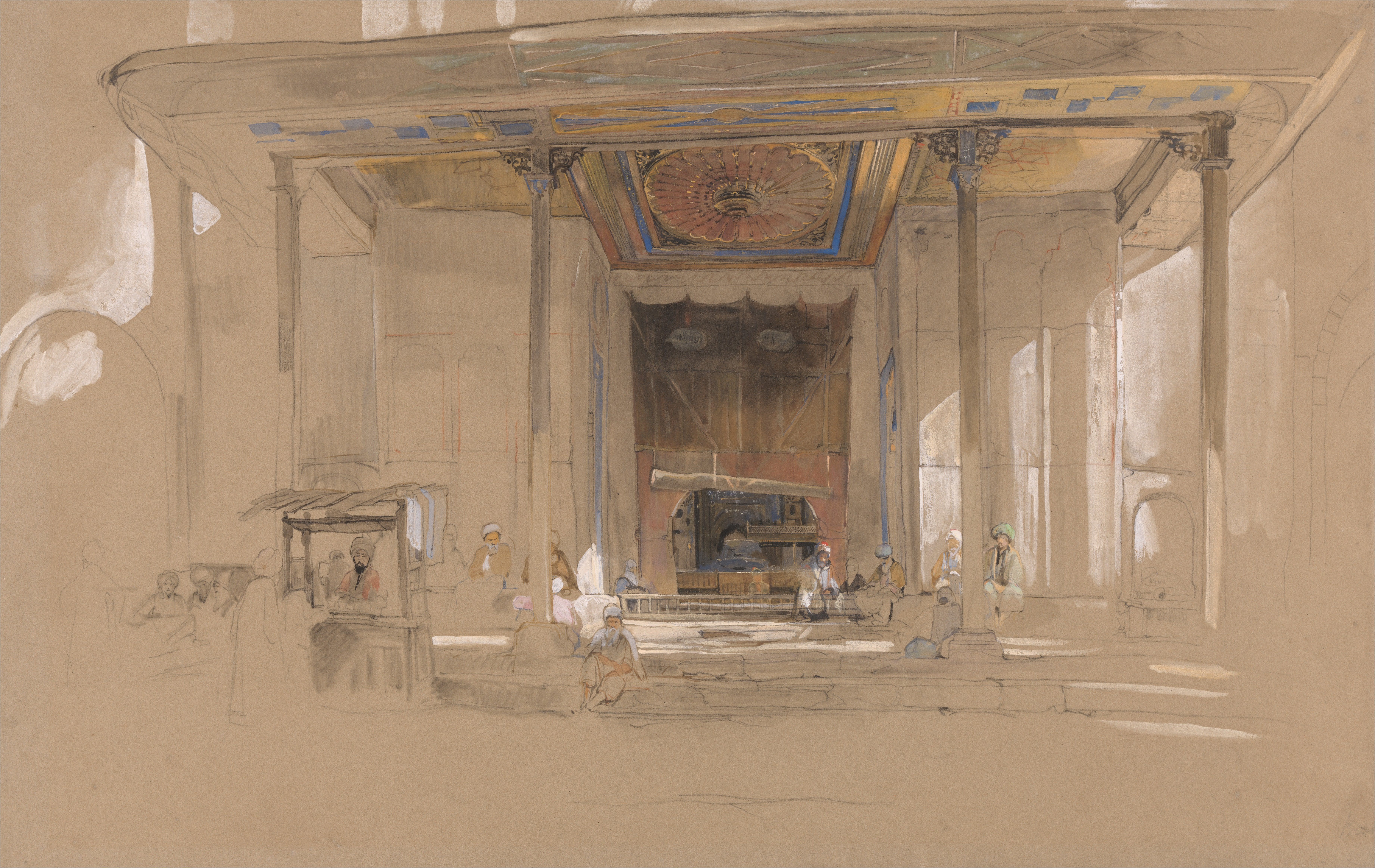The image appears to be a minimalistic depiction of an indoor scene, rendered in very light peach and tan hues, accentuating a feeling of simplicity and subtle elegance. Central to the scene is a large room with sparse details, evoking the atmosphere of an Oriental structure. The composition includes five to seven faintly discernible figures sitting on steps within a vast, covered area. Above these figures, a round design set within a square panel suggests an element of ornate decor, though its specifics remain unclear. 

The foreground is dominated by a dull, light tan expanse, while the background, particularly to the right, hints at natural light filtering through what seems to be a window. Central in the background is a dark-colored curtain, appearing to hang from five noticeable points, which might be nails, suggesting it was hastily or casually attached. There are beams and wooden poles overhead, contributing to the structural feel.

To the right of center, a man sits in what resembles a box-like structure with light streaming in from both sides, possibly indicating windows or openings. Further elements include lightly sketched figures to the left, giving the impression of an unfinished or artistically abstract rendition. The overall aesthetic, perhaps achieved through watercolor or oil paints, imbues the scene with a serene, somewhat dusty ambiance, as if capturing a fleeting moment within a quiet, understated interior.